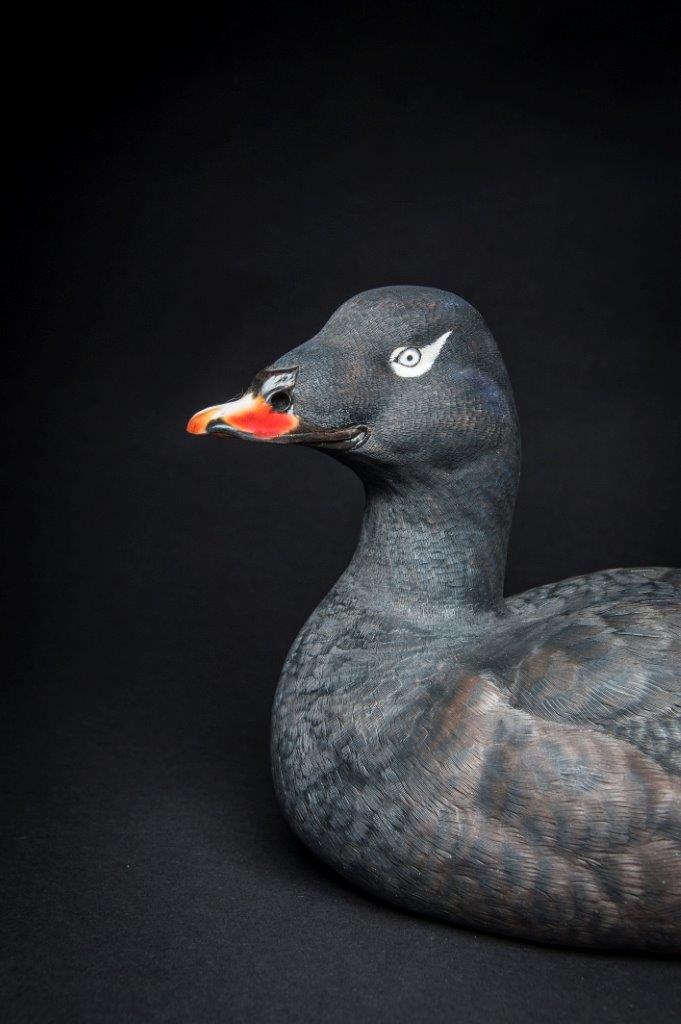In the vertical, color photograph we see the image of a stuffed animal, resembling a duck, set against a pitch-black backdrop illuminated subtly at the bottom. This dark, flat background makes the subject pop distinctly in the frame. The duck appears to be made from a fabric material, giving it a three-dimensional, tactile quality that conveys its nature as a toy. It has a slate gray body with feathers that have subtle hues of pinkish-brown interspersed within them, adding texture and depth. The duck’s beak is predominantly orange, featuring some black accents, while its eyes are stark white, standing out prominently from its face. The overall presentation blurs the line between whether it is a photograph or painting, due to its detailed and lifelike depiction.